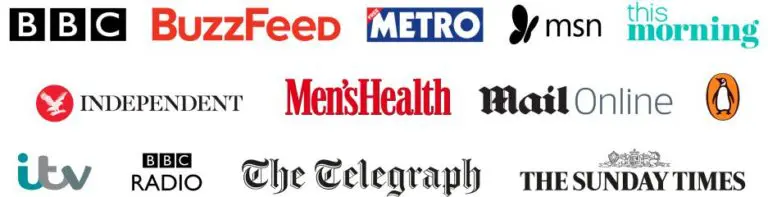The image features a variety of website logos arranged in rows, each distinct and easily recognizable:

Top Row:
1. The logo for BBC showcases big, bold white letters "B", "B", and "C" each within individual black squares.
2. The BuzzFeed logo is displayed in prominent, bold, red letters.
3. The Metro logo features bold, white letters inside a blue box.
4. There is a black butterfly icon paired with the black letters "MSN".
5. The logo for "This Morning" is written in teal letters.

Second Row:
1. A red circle with a bird inside, followed by the word "Independent" in black letters.
2. The Men's Health logo is depicted in bold red letters.
3. The Mail Online logo is present.
4. A penguin inside an orange oval, typically associated with Penguin Books.

Third Row:
1. The ITV logo is written in teal and grayish cursive letters.
2. The BBC Radio logo features the familiar "B", "B", and "C" in black squares above the word "Radio".
3. The Telegraph logo is rendered in a calligraphy-like font.
4. The Sunday Times logo in black letters with an accompanying small drawing above it.